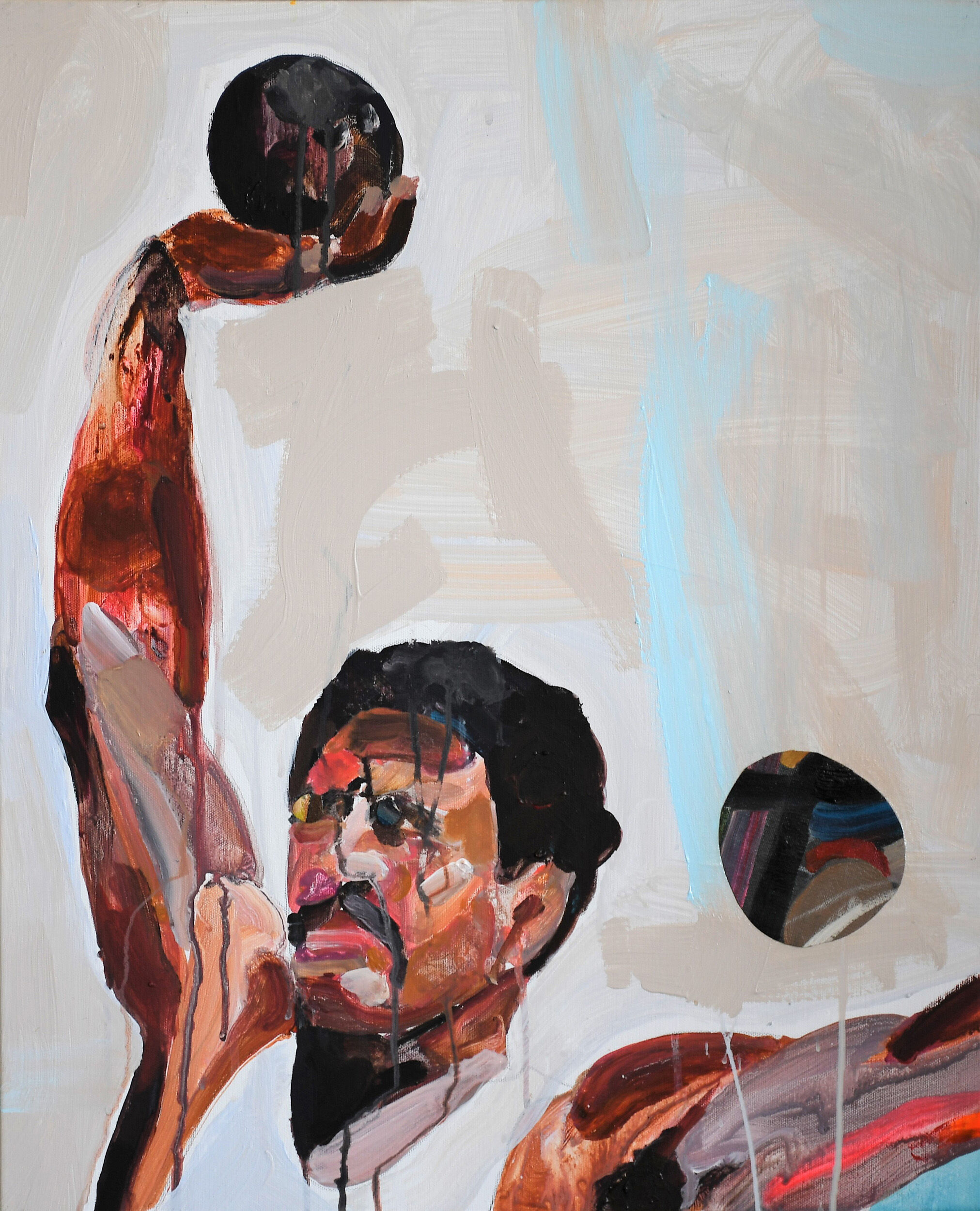This is a detailed watercolor painting of an African-American male athlete engaged in throwing a shot put ball. The man has short black hair and a black mustache, with brown skin tones prominently displayed. His expression is intense, with black paint dripping down his face, adding a raw, dynamic texture that extends down his wrist and arm. He holds a large metal ball in his right hand, which is poised over his head, suggesting the moment before releasing the shot put. The left arm is outstretched and partially out of the frame. The athlete is dressed in a white sleeveless jersey. Additionally, he has a band-aid placed beneath his right eye. His arms feature an intriguing mix of colors, including grays, blues, reds, browns, and blacks, reflecting an abstract artistic style. Various colored streaks, including paint drips, flow from the ball down his hand and along his arm. The background of the painting consists of light white and blue watercolor brush strokes, complemented by a circle motif displaying similar color patterns of black, red, and gray. This semi-abstract piece captures both the physical strength and the painterly expression of the athlete in motion.